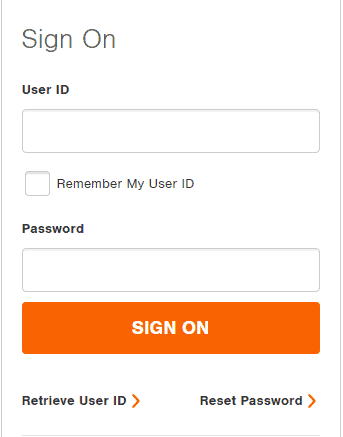Screenshot of a Basic Pop-Up Sign-In Menu

The image captures a screenshot of a simple pop-up menu with a clean design. The background is completely white, accentuated by thin black lines running along the left and right sides of the screenshot.

In the upper left corner, bold large black text reads "Sign On." Just below this, in smaller bold black text, is the label "User ID," under which an empty white rectangular input field is situated. Further down, a small empty white square checkbox is followed by the text "Remember my User ID."

Continuing downward, another bold black label "Password" appears, accompanied by a second empty white rectangular input field directly beneath it. Below this input field, there is a prominent red rectangular button featuring the white text "Sign On."

At the lower end of the menu, the phrase "Retrieve User ID" appears in plain black text at the bottom left corner, next to a small arrow pointing to the right. In the bottom right corner, bold black text "Reset Password" is displayed, accompanied by another right-pointing arrow.

A thin black line at the very bottom of the screenshot signifies the end of the pop-up menu content. This simple and clean design serves as a straightforward sign-in interface for an unspecified app.